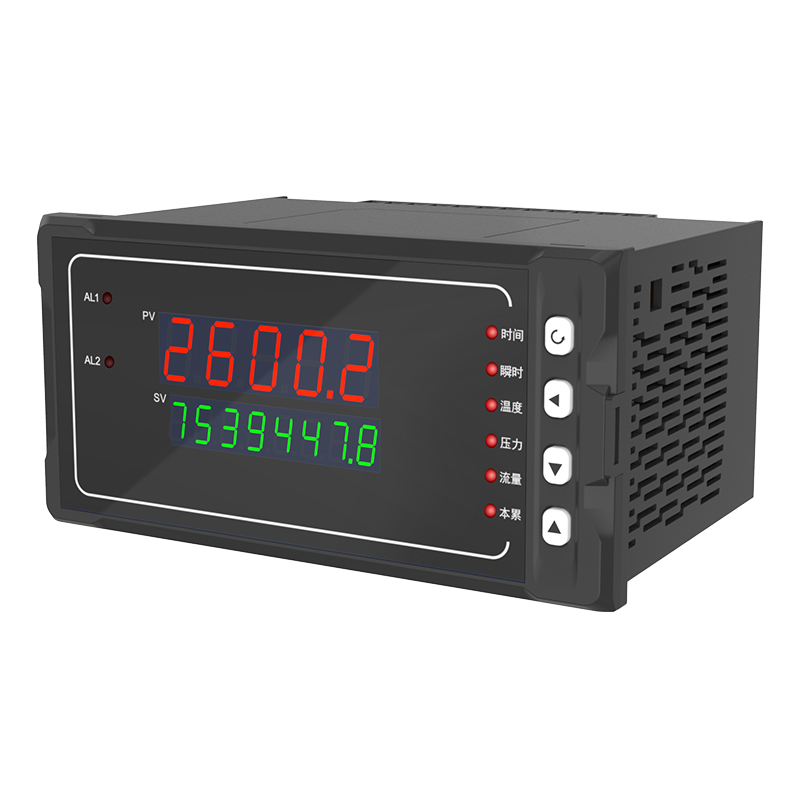The image depicts a digital meter, an electronic device set against a white background due to the photo editing that removed its original context. The device itself is a large, gray, rectangular "black box" with its front panel facing southwest, revealing its front and right sides. On the right side, there are multiple small, rectangular cut-out shapes, suggesting ventilation or access points.

The front face of the meter prominently features a digital display encased within a white frame. On the upper left, the labels "AL1" and "AL2" are inscribed, each accompanied by a small circular indicator—AL1 has a red dot, and AL2 has a black dot, though neither is currently illuminated. Centrally located on the display is "PV2600.2" written in red digital numerals, while directly below it, in green, is "SV7539447.8." 

At the lower portion of the device, there are four white control buttons arranged vertically. The topmost button resembles a rewind symbol (a half-circular arrow), followed by a triangle pointing left, another triangle pointing down, and the last triangle pointing up. Additional features include some Chinese writing on the right side and various other lights and indicators, potentially capable of illuminating red.

The equipment’s styling reflects Photographic Representational Realism, offering a detailed and true-to-life depiction of its structural and functional elements.